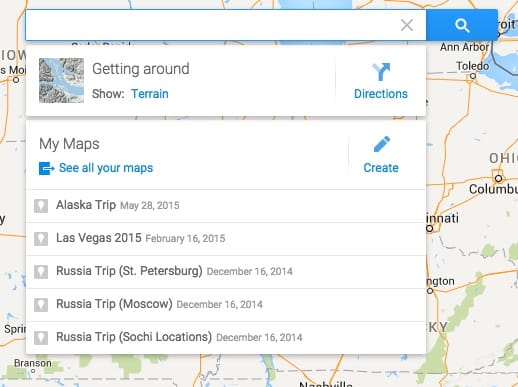This image is a screenshot from a mapping website or app, featuring a schematic map of Ohio and its surroundings. In the background, the names of various locations are visible, including "Ohio," "Columbus," "Cincinnati," and "Toledo." At the top, "Ann Arbor" in Michigan is also marked, as well as some areas of Kentucky.

The focus of the image is on two white interface boxes that partially obscure the map. The first box is titled "Getting Around" and includes options like "Show Terrain" and "Directions," allowing users to view the terrain or get route information. Below this, the second box is titled "My Maps," offering options to "See All Your Maps" or "Create" a new map. Additionally, it displays a list of five previously created maps:

1. "Alaska Trip" from May 28th, 2015
2. "Las Vegas, 2015" from February 16th, 2015
3. "Russia Trip, St. Petersburg" from December 16th, 2014
4. "Russia Trip, Moscow" from December 16th, 2014
5. "Russia Trip, Sochi locations" from December 16th, 2014

Overall, the screenshot provides a glimpse into the interface and functionalities of the mapping tool, highlighted by specific locations and user-generated maps.